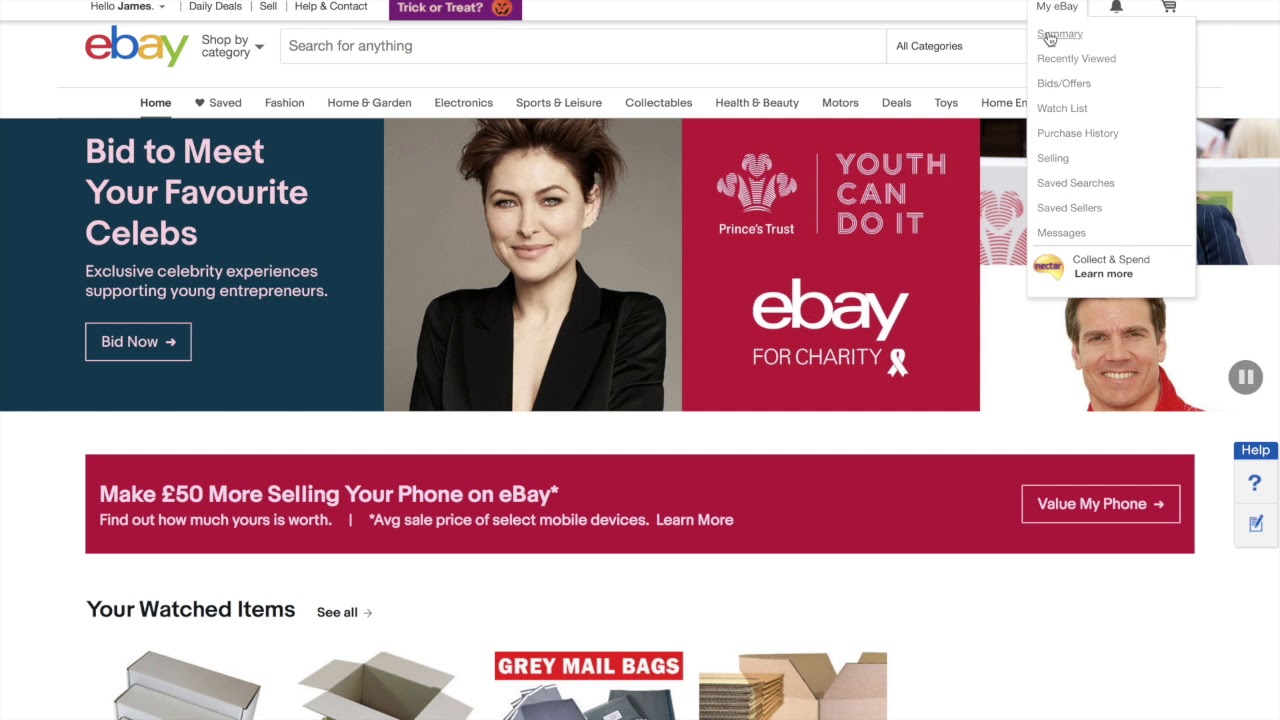The image depicts a cluttered eBay webpage interface. In the top left corner, there is a small, blurry text which appears to say "Hello James." Just below, a purple box with a pumpkin jack-o-lantern design reads "Trick or Treat." Below this box, the iconic red, blue, yellow, and green eBay logo is prominently displayed along with the phrase "Shop by Category." A search bar labeled "Search for Anything" is centrally located, alongside a drop-down menu titled "Categories."

In the top right corner, a tab labeled "My eBay" is visible, with its drop-down menu currently expanded. On the left side of the page, a dark gray box contains the text "Bid to Meet Your Favorite Celebrity, Exclusive Celebrity Experiences Supporting Young Entrepreneurs," accompanied by a square button labeled "Bid Now." Underneath, a burgundy rectangular advertisement announces "Make £50 More Selling Your Phone on eBay," with a nearby square button labeled "Value My Phone."